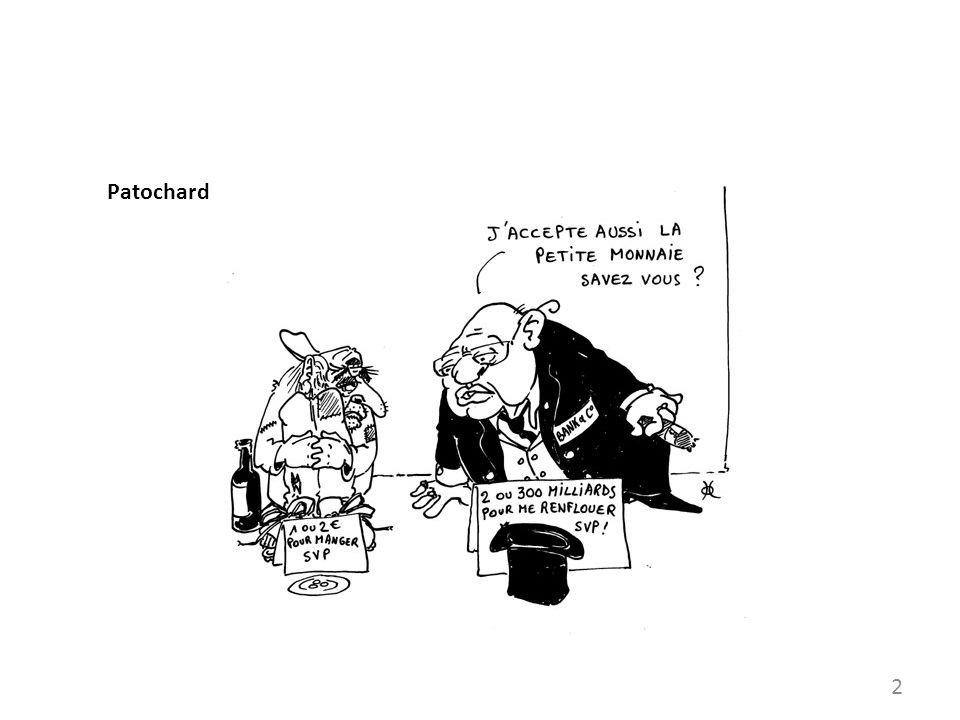This black-and-white caricature cartoon, titled "Patochard" in the upper left corner, portrays two men sitting on the ground, each with a sign written in French. The man on the left, likely homeless, hugs his knees to his chest and wears a backward cap. Beside him is a dark bottle with a bright label. In front of him, a small flat plate holds three coins, hinting at his destitution. His sign includes the phrase "A-O-2-E Poor Manager S-V-P." Next to him, an older, balding man, possibly a banker, dons glasses, a dark suit with a tie, and a jacket bearing a "Bank of C" patch on the upper left lapel. He holds a cigar and has his top hat placed upside down on the ground, accompanied by a sign stating "2-0-300 Milliards Poor Me Renflower S-V-P." This satirical image likely appeared in a magazine or newspaper, emphasizing a humorous yet poignant comparison of their social statuses.